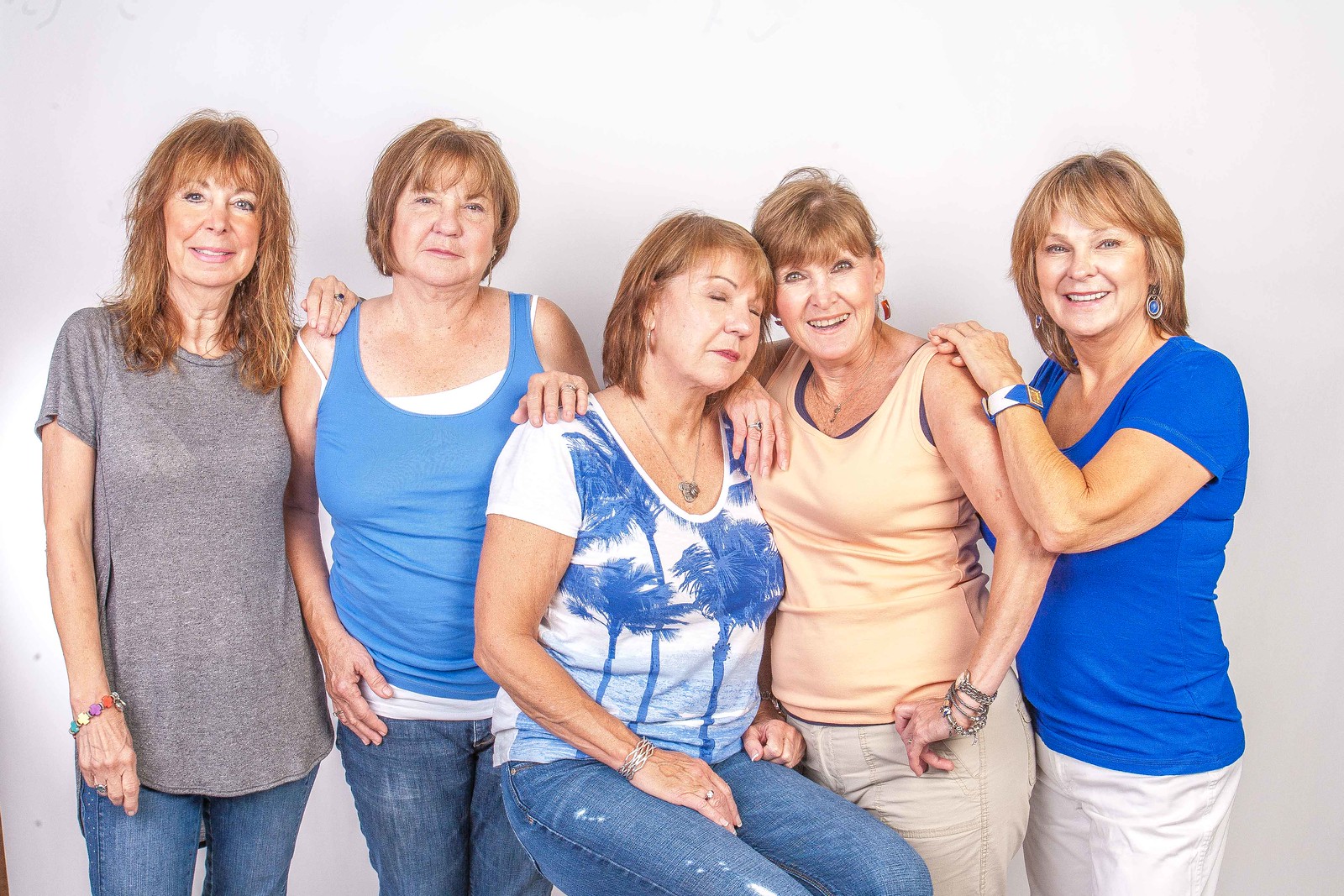This photo features five middle-aged to older women, possibly in their 60s, who appear to be related due to their strikingly similar appearances. Their hair, varying from chin-length to shoulder-length, is a reddish-brown or orangish-brown hue. The background is a light orchid color with a white light illuminating it, making the picture very bright and well-lit. The women are dressed in summery outfits; some wear tank tops and others t-shirts, mostly in shades of blue, beige, and gray. Four of the women are wearing blue jeans, while the woman in the middle, who is seated with her eyes closed and facing to the right, has on a white t-shirt with a blue palm tree graphic and blue jeans. Her hands rest on her lap. The woman on her immediate left wears a gray t-shirt, and next to her is another woman in a blue tank top. To the right of the seated woman, one wears a tan or orange tank top and the other a blue short-sleeve t-shirt. They are all smiling, adding a warm, familial touch to the scene. The overall color theme is very blue, and their close physical proximity and similar features, like their hair color and casual, coordinated outfits, suggest that they are either sisters or very close friends.